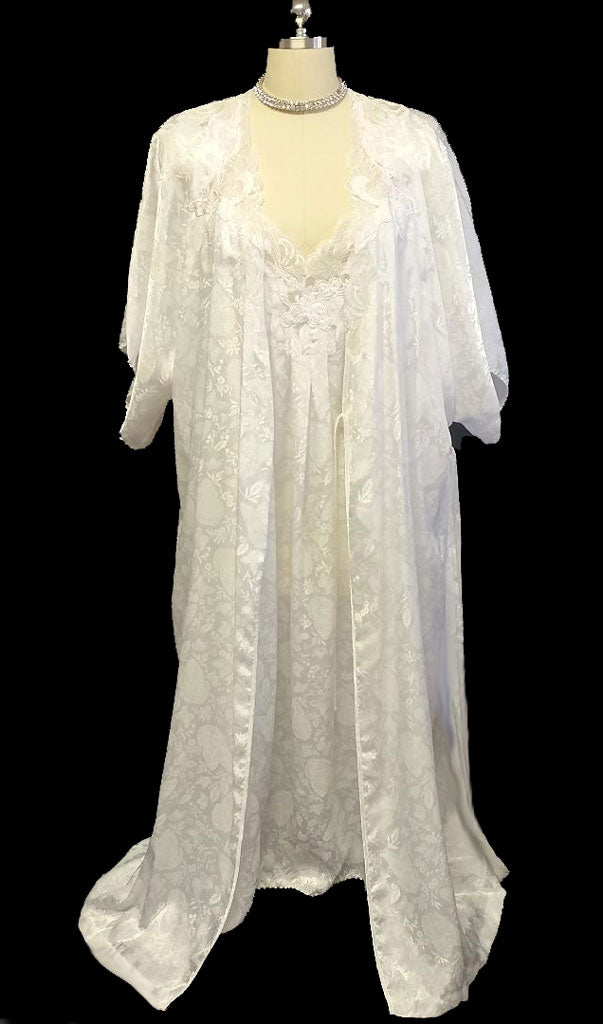This indoor color photograph captures a vintage-style, white lace nightgown and robe set displayed on a headless and armless cream fabric mannequin. The mannequin, which has a silver ball at the top of its neck area, is adorned with a double-layered, diamond-like choker necklace. The background is stark black, drawing attention to the intricate details of the gown. The elegant set, possibly intended for a wedding night, features a sheer, satin fabric with a faint floral and leaf design imprinted on it. The gown has short sleeves and flows down gracefully to the floor. The robe, which complements the nightgown, also features lace detailing around the neckline and has three-quarter sleeves. This display, which could be part of a museum exhibit, highlights the delicate and ethereal quality of the garments.